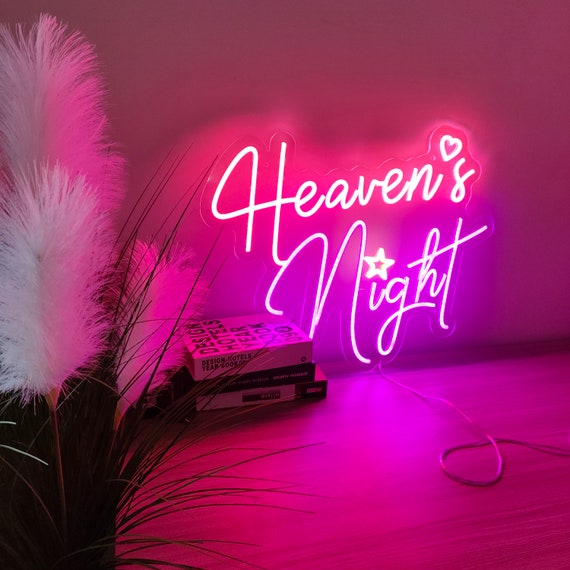The photograph captures an indoor scene highlighted by a vibrant neon light sign that reads "Heaven's Night." The word "Heaven's" is depicted in neon pink with a heart symbol in place of the apostrophe, while "Night" is in neon purple featuring a yellow star over the 'i'. This neon sign, mounted on the wall, casts a pink and purple glow across the room. The area around the sign is clear, making the light's plug visible as it loops forward and exits to the right.

The lower portion of the wall meets a floor made of horizontal slatted wood, resembling linoleum. In the bottom left corner, three delicate strands of white pompous grass emerge from a small black rectangular base. To the right of this grass, directly under the sign, three books are stacked: the top book is Zion Hotel's Yearbook, 090, followed by a black-covered book and another with a white cover. The combined elements of neon lighting, wood flooring, eclectic books, and decorative pompous grass create a visually striking and cozy indoor atmosphere.